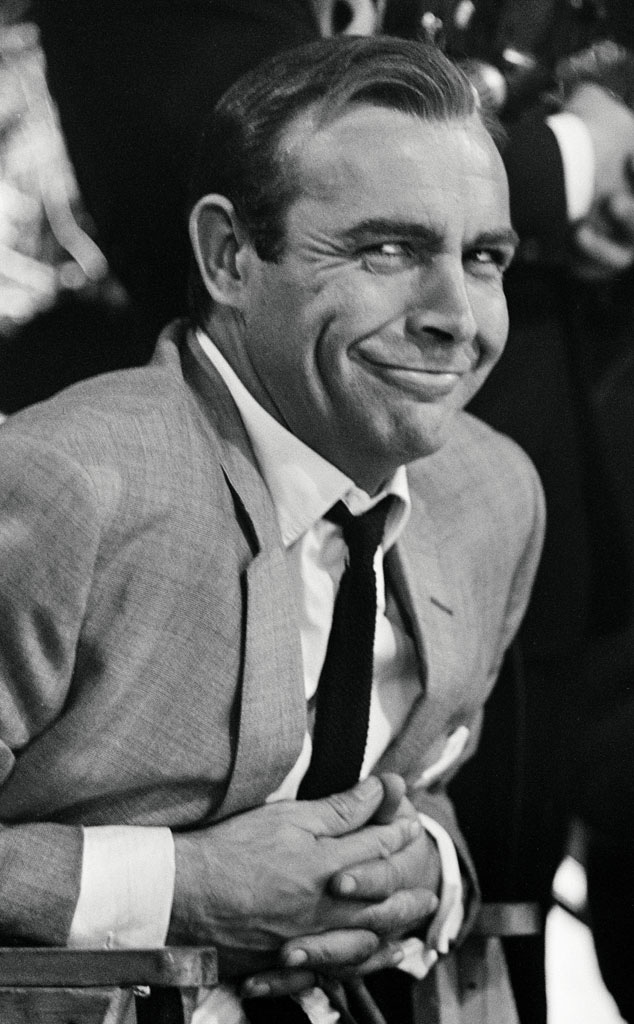The black-and-white photo, taken in 1964, captures a man who bears a striking resemblance to Sean Connery, if not the man himself. He is seated and leaning slightly over the wooden arms of a chair. The image offers a close-up profile of his right side, turning slightly towards the camera, revealing his dark, wavy, short hair styled in a manner reminiscent of the 1960s. His eyes crinkle in a slight smile or smirk, marked by distinct crow's feet. He is dressed in a light gray, linen-like suit jacket with white cuffs peeking out from the sleeves, and his hands are clasped together in front of him. He completes the look with a slightly loosened black tie over a white collared shirt. The background is blurred, featuring people in dark suits, adding to the focal emphasis on the man.